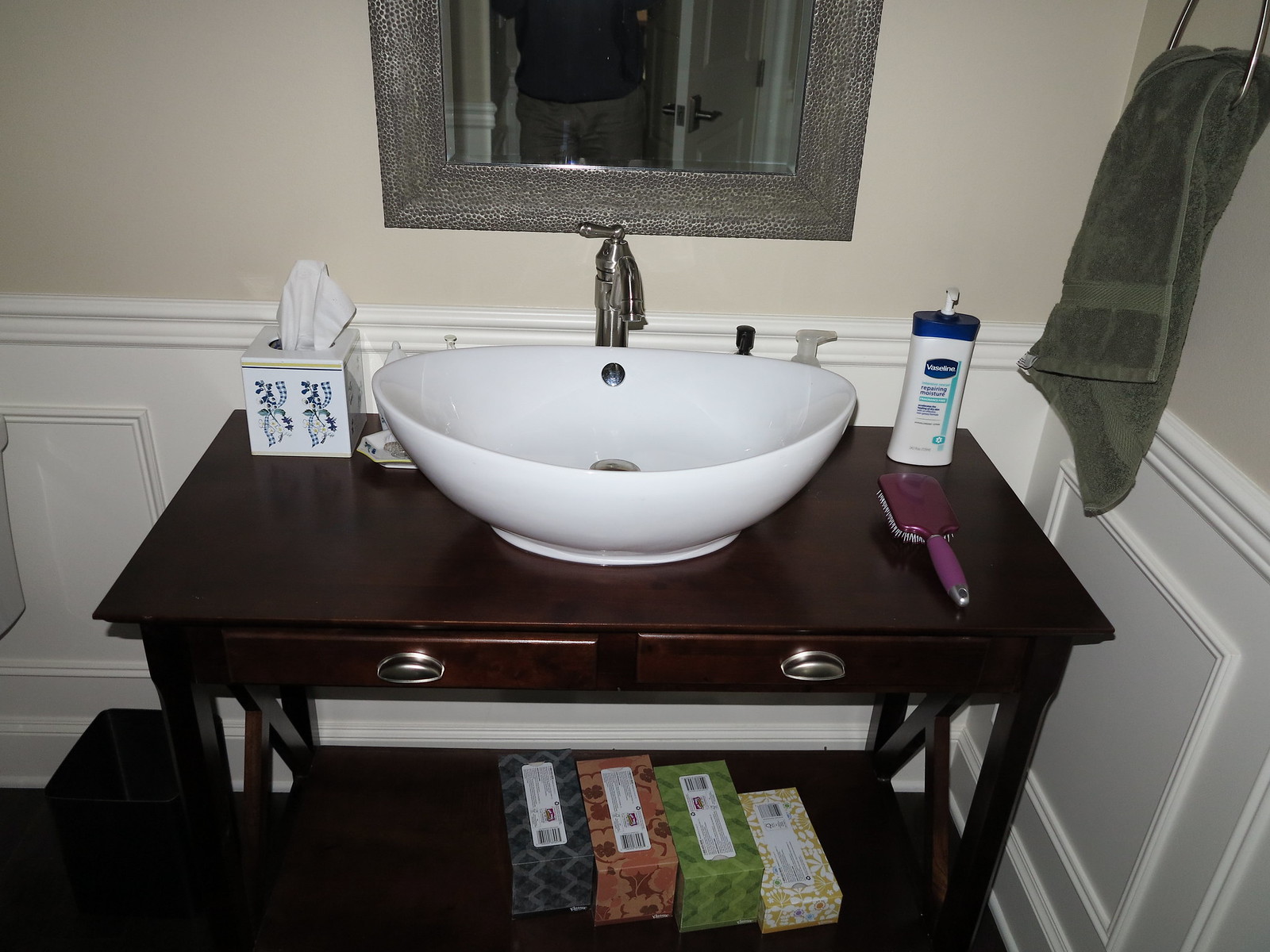This image showcases a meticulously arranged desk set against a dual-tone wall, with the lower portion painted white and the upper part in a cream shade. A silver-framed mirror prominently hangs above the desk, adding a touch of elegance. Adjacent to the mirror, a green towel is neatly draped over a silver towel rack on the right.

The desk itself is crafted from rich mahogany wood, presenting an auburn hue. It features a large, gleaming white ceramic sink fitted with a modern silver faucet. To the right of the sink, a purple hairbrush lies next to a rectangular white and blue shampoo bottle. On the left side of the sink, a box of tissues provides practicality.

Beneath the desk, there are four additional tissue boxes neatly arranged in a row, displaying various colors: gray, orange, green, and yellow. The desk also boasts two silver handles on its front, offering functionality and ease of access to any stored items within.

The wall's division is ingeniously aligned with the silver faucet, creating a harmonious alignment that extends horizontally to the right.